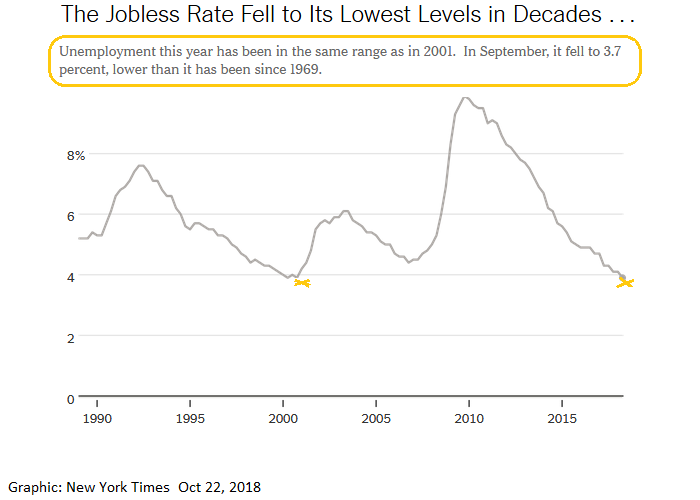This infographic, attributed to the New York Times and dated October 22, 2018, is titled "The Jobless Rate Fell to its Lowest Levels in Decades." Below the title, a subheading enclosed in a yellow rectangle states, "Unemployment this year has been in the same range as in 2001. In September, it fell to 3.7%, lower than it has been since 1969." The chart features a line graph with unemployment rates plotted from 1990 to 2018, with the x-axis marked in five-year increments and the y-axis detailing percentages from 2% to 8%. Notably, the graph highlights significant unemployment rate drops below 4% in 2001 and shows a gradual decline reaching 3.7% around 2018, following a peak in 2010 and a gradual decrease starting from 2016. The data visualization effectively underscores the historical context of unemployment trends over nearly three decades.